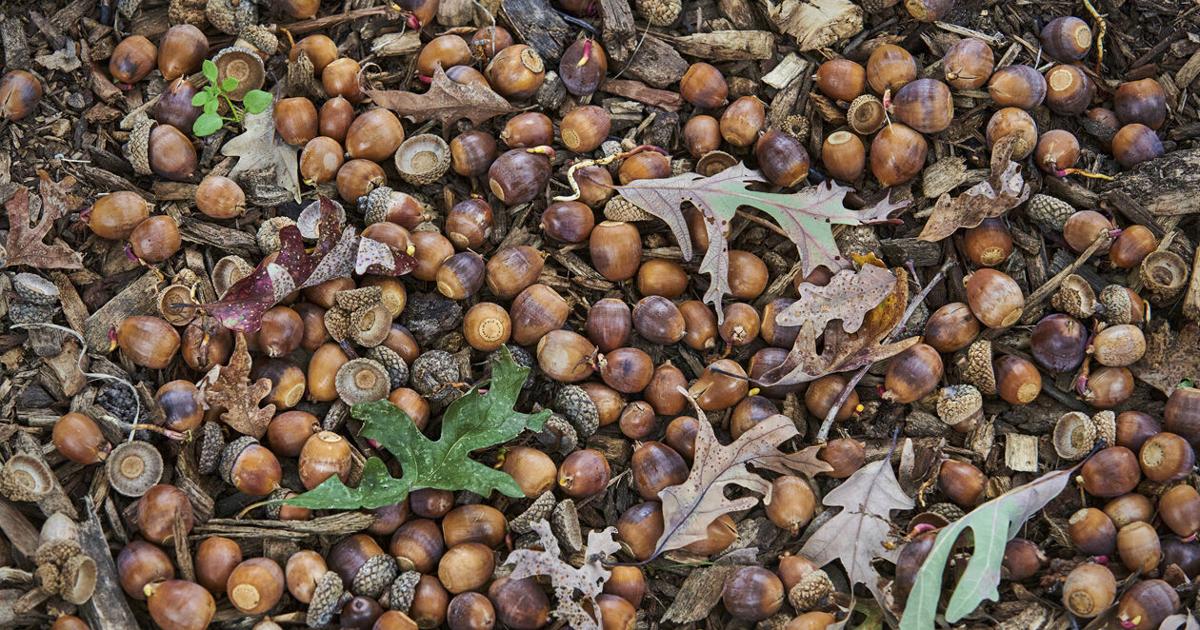This professional, highly detailed color photograph captures a wide-angle view directly downward onto a forest floor, teeming with acorns. The scene, predominantly in shades of rusty brown and golden hues, vividly illustrates the essence of fall, with the ground almost completely carpeted by an uncountable number of acorns and their tops. Scattered among the acorns are a mix of leaves, predominantly brown and shriveled, but punctuated by occasional green leaves and a single red one, hinting at a seasonal transition. The acorns exhibit a spectrum of colors from light chestnut and tan to darker brown and even black. The ground beneath them appears grey and barren, with a bit of dead foliage interwoven beneath the acorns. There are patches within the image where the acorns' colors seem to reflect a purplish tinge. No writing or extraneous objects disrupt the focus; the image is purely a medley of natural elements, concentrated in the center but tapering off slightly towards the corners, encapsulating an intricate and immersive forest floor tableau.